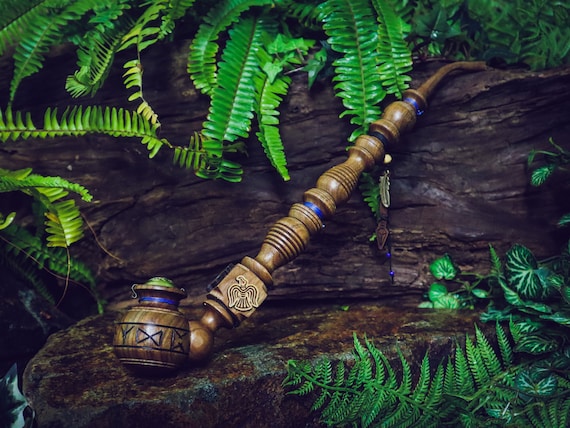The detailed close-up image showcases an intricately designed smoking tobacco pipe, made primarily out of wood with distinct blue segments and adorned with what appear to be Nordic or Norse symbols. This stylish and rather regal pipe features golden accents and various intricate patterns, adding to its luxurious look. The pipe, with a spherical top part inscribed in black and a neck portion encircled by a blue ring, rests upon a rustic piece of bark. This bark is surrounded by green grass, colorful petals, and a few wet rocks, giving the scene a fresh, natural appearance. The background suggests a well-lit, designer park setting, free from any other noticeable objects, people, or text. The image is colorful and crystal clear, highlighting every meticulous detail of the pipe and its surroundings.